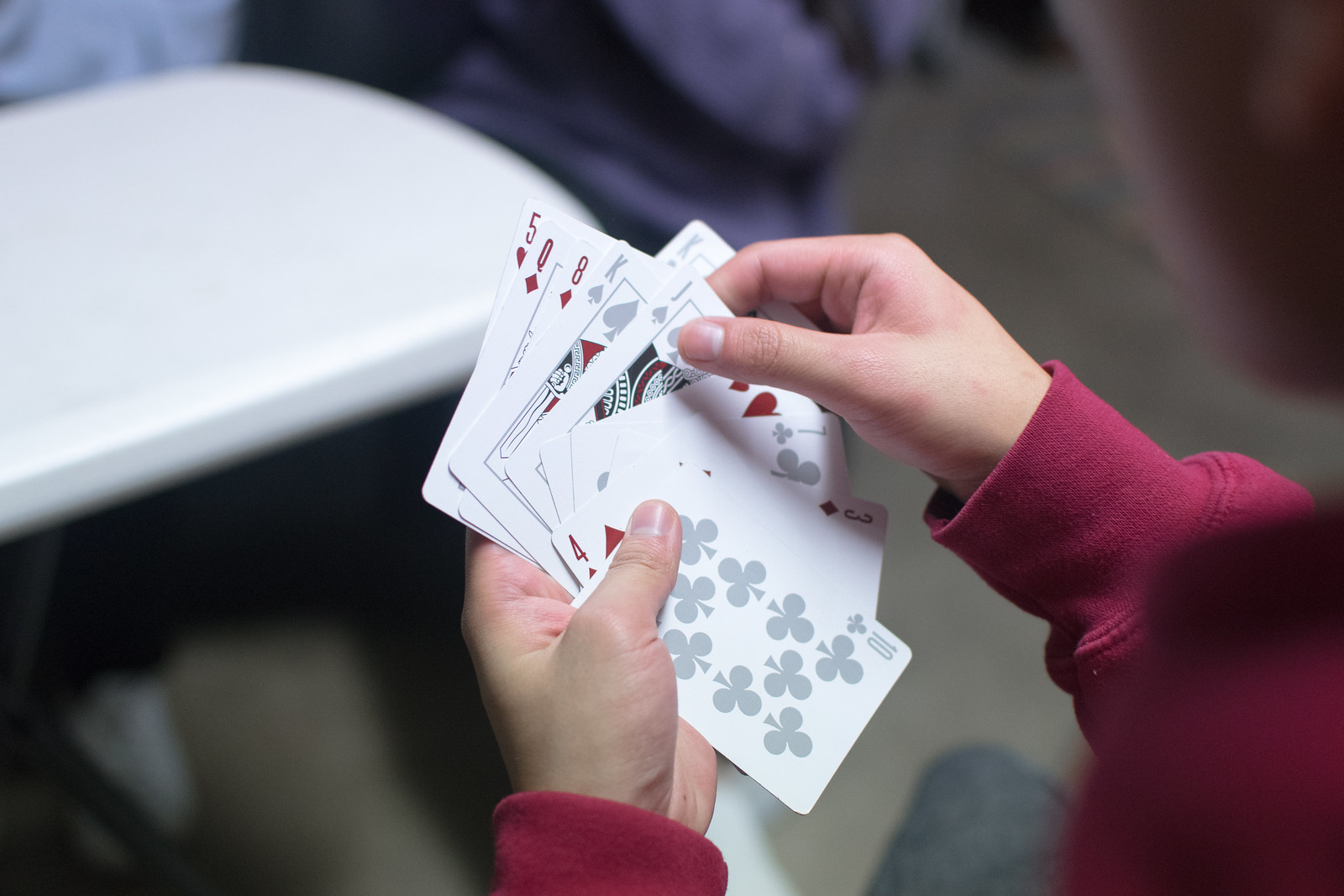A person, clad in a red long-sleeved sweater, is captured in the midst of a card game. They hold a diverse hand of playing cards in their left hand, expertly fanned out to reveal the faces. The hand consists of a five of hearts, queen of diamonds, eight of diamonds, king of spades, seven of clubs, three of diamonds, and ten of clubs. The individual is in the process of removing the jack of spades with their right hand, delicately grasping it between their thumb and forefinger. In the blurred, out-of-focus background, a white card table is faintly visible, suggesting an ongoing game. The focus and detail highlight the tension and strategy involved in the moment.